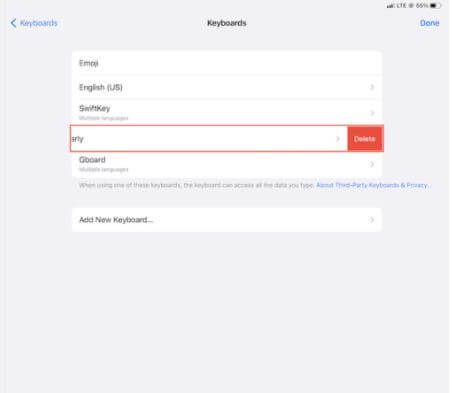The image displays a white background featuring a smartphone screen with the "Keyboards" settings open. At the top, a blue bar reads "Keyboards," accompanied by a black back arrow to the left and a blue "Done" button to the right. The battery indicator shows 84%, and there are three bars of signal strength.

Below the title "Keyboards" in bold black text, the screen lists various keyboard options. The first option is "Emoji," followed by "English (US)," both in black text. Next is "SwiftKey" with a forward arrow indicating additional settings. 

Further down, a red search box with the letter "Y" typed inside is present, alongside a red delete button. Beneath these, the "Gboard" option appears with a brief description. The last item on the screen is "Add New Keyboard," which includes a forward slash for additional settings.

The clickable elements, such as "English (US)" and "SwiftKey," signify that users can modify these settings by selecting them. The overall interface provides a clear and structured view of the available keyboard options and settings.